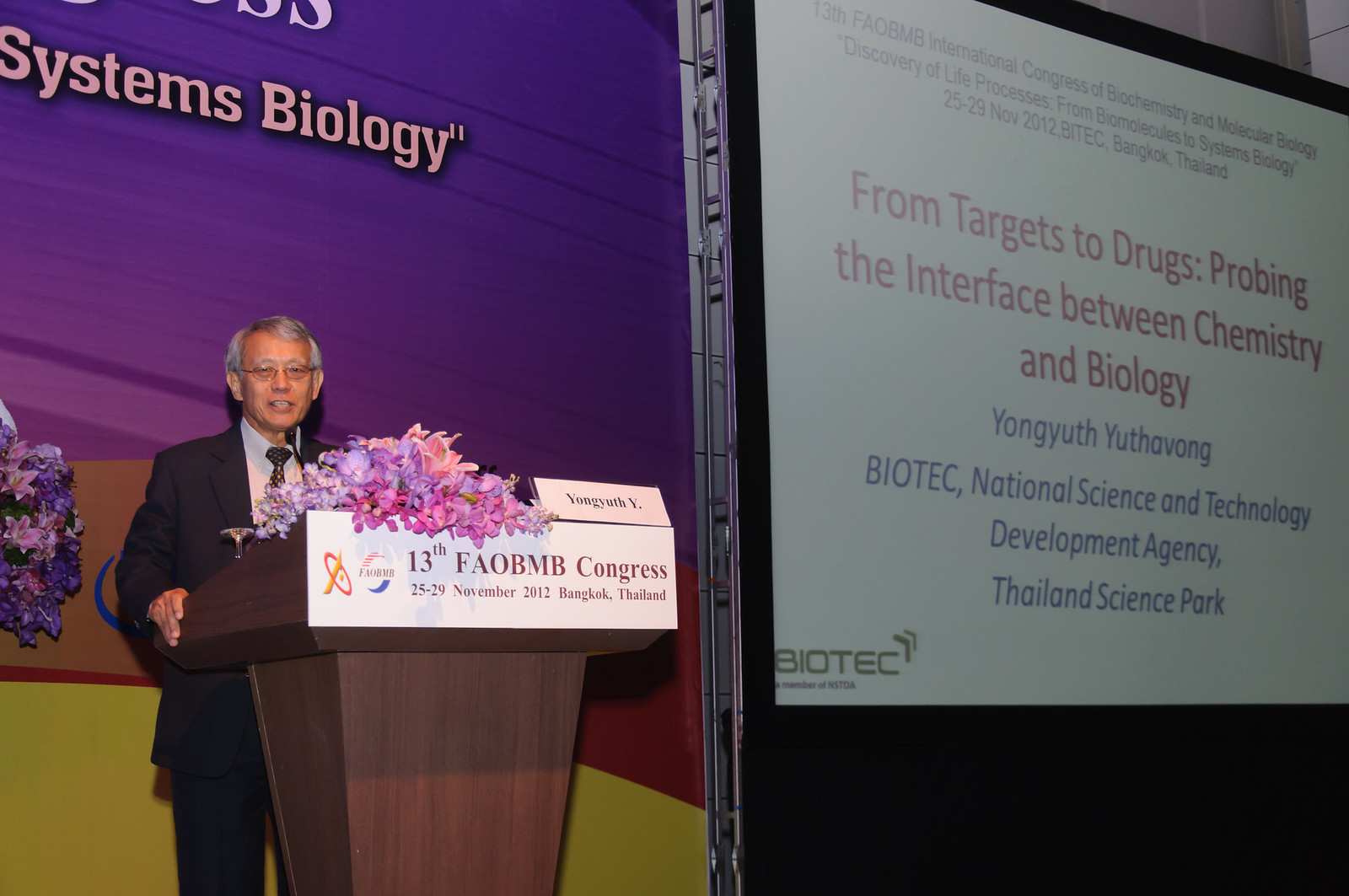This photo captures an elderly Asian man with gray hair and glasses, standing on the stage of a conference or seminar set in Bangkok, Thailand. Dressed in a black suit, white shirt, and black tie, he is speaking from behind a wooden podium adorned with purple flowers. The podium bears a white sign reading "13th FAO B.N.B. Congress" along with the dates "25th to 29th November". The stage backdrop is divided into two colorful sections: a purple section on the left with "Systems Biology" emblazoned above the speaker’s head, and a white section on the right displaying "From Targets to Drugs: Probing the Interface Between Chemistry and Biology". Beneath the text, it lists the name Yong Yusha Hong and the affiliation "Biotech, National Science and Technology Development Agency, Thailand Science Park", with a Biotech logo. The man stands slightly to the left side of the image, facing forward, providing a focal point amidst the detailed and informative background.